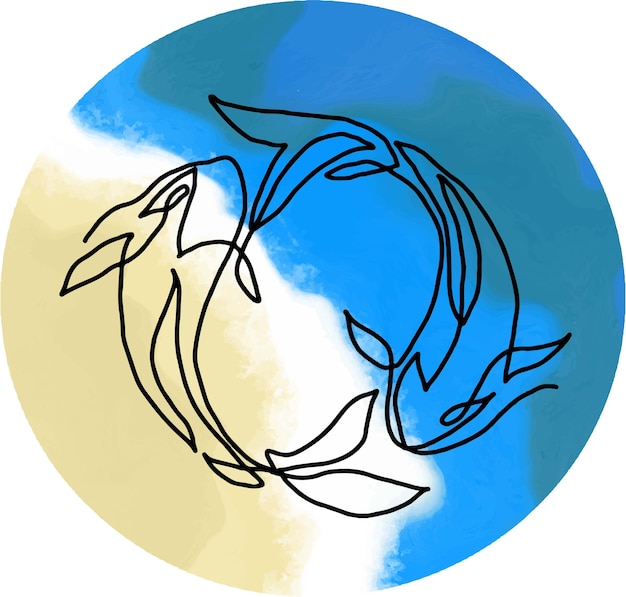The image depicts a digitally crafted artwork resembling a globe, characterized by its bright, vivid colors and harmonious composition. The top left section of the globe features shades of turquoise blue with accents of green, suggesting ocean and land elements. A diagonal band of white slices through the center, transitioning into a tan or beige hue on the opposite side, creating a visual effect as if the globe is tilted slightly. At the heart of this scene are two black line-drawn fish, arranged nose to tail and tail to nose, forming a continuous yin and yang-like circle. This arrangement also mimics the motion and balance of the yin-yang symbol, emphasizing harmony within the colorful background of blue, muted green, white, and tan. The black-outlined fish encircle the central white section, reinforcing the theme of interconnectedness and balance in the artwork.